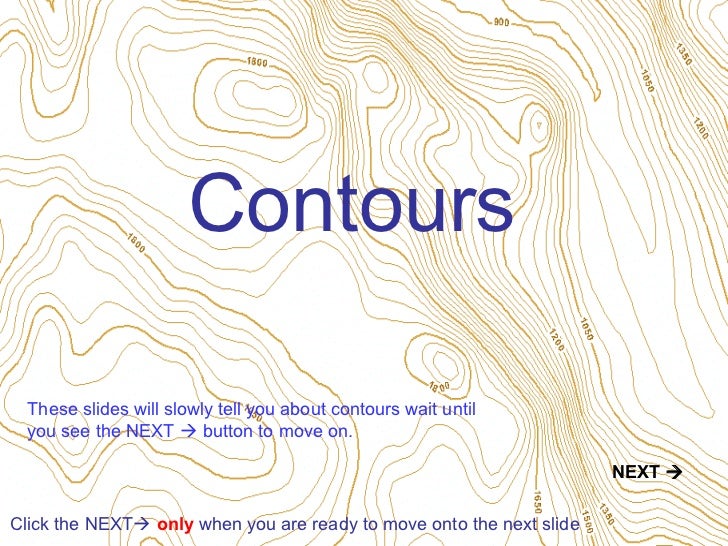The image is a rectangular diagram resembling a topographical map, with a white background. Dominating the center is the word "Contours," written in dark blue text with a capital 'C'. Below this, a series of instructional text reads, "These slides will slowly tell you about contours. Wait until you see the next arrow button to move on. Click the next arrow only when you are ready to move on to the next slide."

The illustration features gold and dark brown contour lines, meticulously tracing the elevations of an unspecified terrain. The lines vary in spacing, becoming closer together in some areas and farther apart in others, indicating changes in elevation with numbers like 1200 and 1050. This arrangement creates a 3D effect, emphasizing the depth and contours of the land. At the bottom of the image is a small, clickable "next" arrow, guiding viewers to proceed once they are ready to move to the next slide. The combination of detailed contour lines and instructional text provides a step-by-step tutorial on understanding the landscape’s topography.